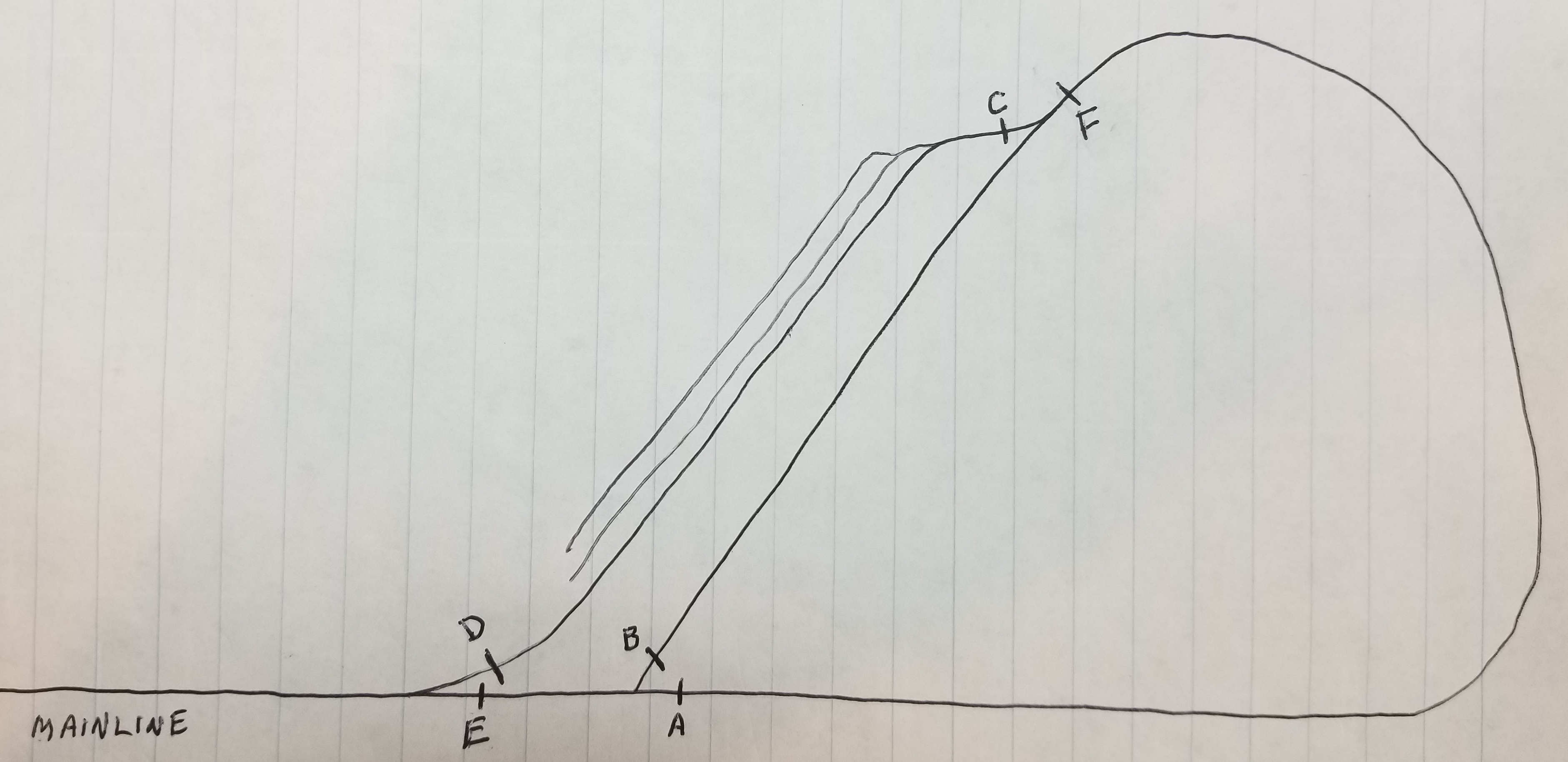The image depicts a detailed diagram sketched on lined paper, where the lines are barely visible in a faded gray. The paper displays a gradient, starting with a bluish hue in the center and transitioning to a peach color on both the right and left edges. In the illustration, a prominent horizontal line labeled "main line" runs from left to right. This line features a segment that curves upward then downward, reconnecting with the initial horizontal line. Below this main line, multiple shorter lines branch out, some at an angle and labeled with letters. The diagram includes the following labeled points: "D" with a dash, "E" with a dash beneath it, "B" with a dash next to it, "A" with a dash beside it, "C" with a dash above it, and "F" also with a dash above it. Notably, the two leftmost lines do not reconnect with the main line, unlike the others. The intricate details and color variations of the paper enhance the overall presentation of the diagram.